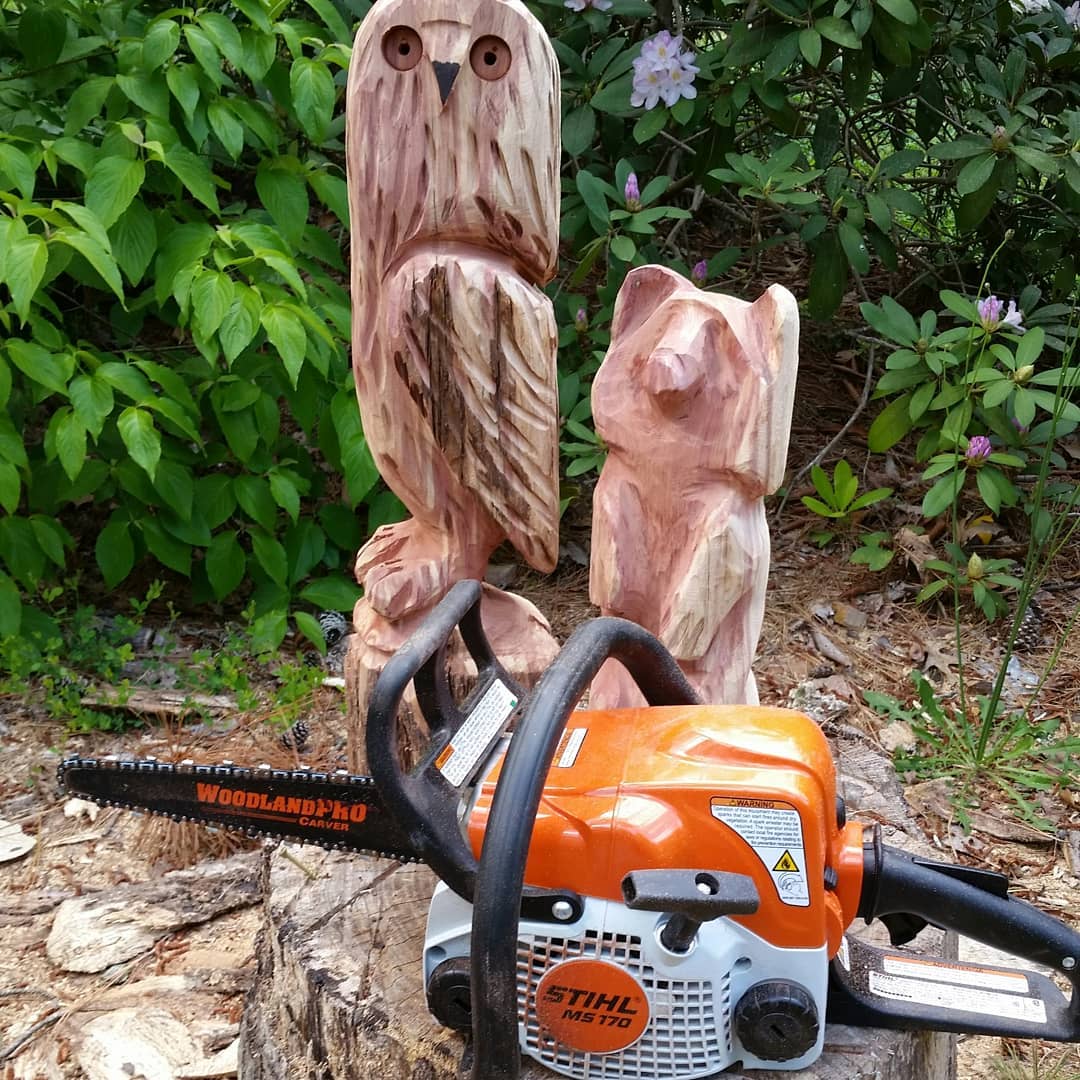In a sunlit outdoor setting, an orange and black STIHL chainsaw rests against a wooden carving of an owl and a bear. The chainsaw, featuring the name "Woodland Pro" in orange letters on its black blade, appears to have been used to create these intricate sculptures. The bear, standing on its hind legs with front paws in front, and the owl, perched on a stump, stand prominently as decorative figures. Behind these carvings, lush green plants and blooming purple flowers fill the background, enhancing the scene's natural beauty. The detailed craftsmanship of the owl's hollowed eyes and the bear's distinct nose and paws are clearly visible, adding character to the wooden figures. The entire scene is well-lit, with no significant shadows, showcasing the vibrant and lively outdoor environment.